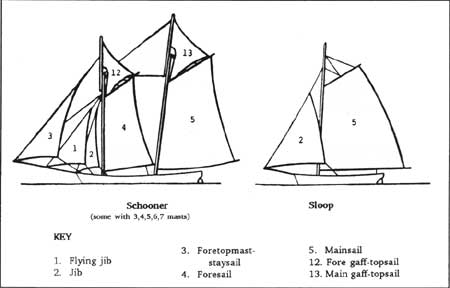This image features a black-and-white line drawing of two types of sailboats— a schooner and a sloop—against a white background, resembling illustrations from an old textbook. The schooner, depicted on the left, is the larger vessel with more sails and is annotated with numbers 1, 2, 3, 4, 5, 12, and 13 that correspond to various parts of the sails. The sloop, a smaller boat on the right, has fewer sails. Below the schooner, the label indicates "schooner," with a note in quotations about possible configurations with 3, 4, 5, 6, and 7 masts. Similarly, the term "sloop" is written beneath the smaller boat. A key beneath the illustrations details the sail parts: 1 is the flying jib, 2 is the jib, 3 is the foretopmast staysail, 4 is the foresail, 5 is the mainsail, 12 is the foregaff topsail, and 13 is the maingaff topsail. This detailed visual aid allows viewers to learn and identify the different components of sails on these traditional sailing vessels.